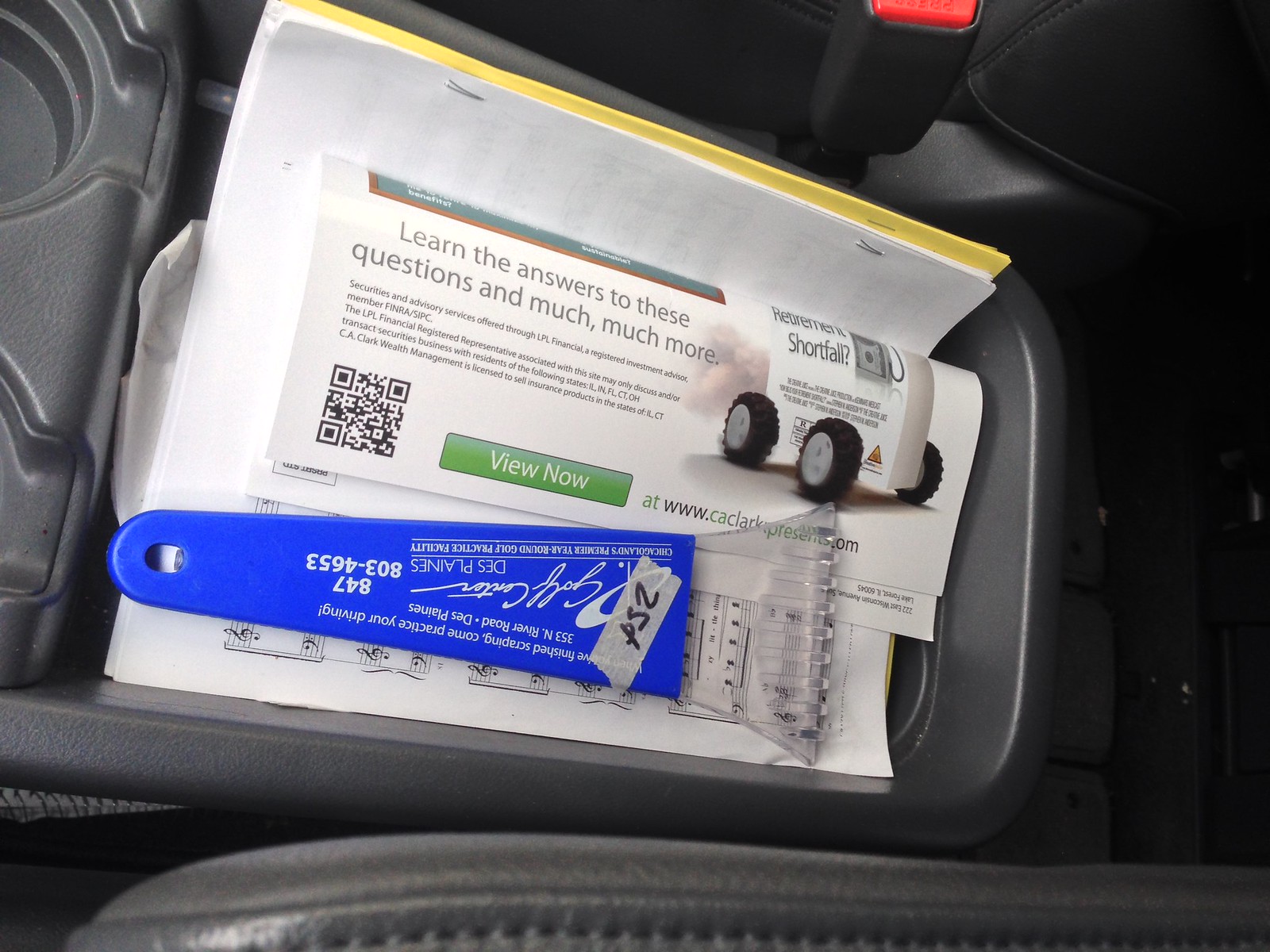This image captures the inside of a well-maintained vehicle, specifically the console between the two front seats. The dark gray leather interior exudes a sleek and clean look. Within the open console, there is an assortment of items, including a blue plastic ice scraper, which appears to be a promotional item from "Chicagoland's premier year-round golf practice facility." A piece of tape on the scraper reads "25 cents," hinting that it may have been purchased at a garage sale. The glove compartment also holds a variety of papers, including a folded pamphlet discussing economic topics, sheet music stapled together with other documents, and a conspicuous yellow paper with the headline "Learn the answers to these questions and much, much more," accompanied by a QR code linked to CA Clark's website. The vehicle's interior is notably clean, with visible cup holders and the edge of the seat belt buckle area enhancing the overall detail of the scene.